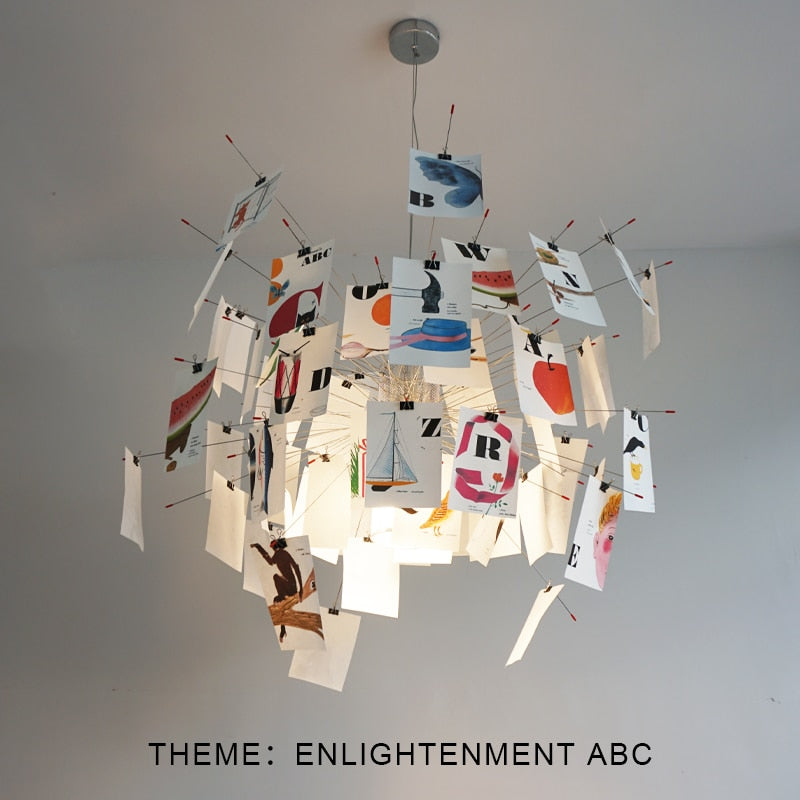The image depicts an intricate mobile hanging from a white-ceilinged room, which also functions as a light fixture. The mobile, titled "Theme: Enlightenment ABC," is composed of numerous flashcards, each attached to metal rods or wires extending from a central lamp structure. This lamp not only serves as the core of the mobile but also illuminates the cards, casting light from behind them. The flashcards bear a variety of alphabet letters and corresponding images, such as a bee, a bird, a hammer poised to hit a blue hat, a sailboat, an apple, a nest, a monkey in a tree, a drum, and a watermelon. Letters highlighted include A, B, C, D, N, R, W, and Z, with creative illustrations like a ribbon-wrapped R and an ABC sequence featuring a cat head within the letter C. The square photograph captures this educational and artistic fixture against a gradient gray background, emphasizing the illuminated and cleverly arranged cards that encircle the lamp.